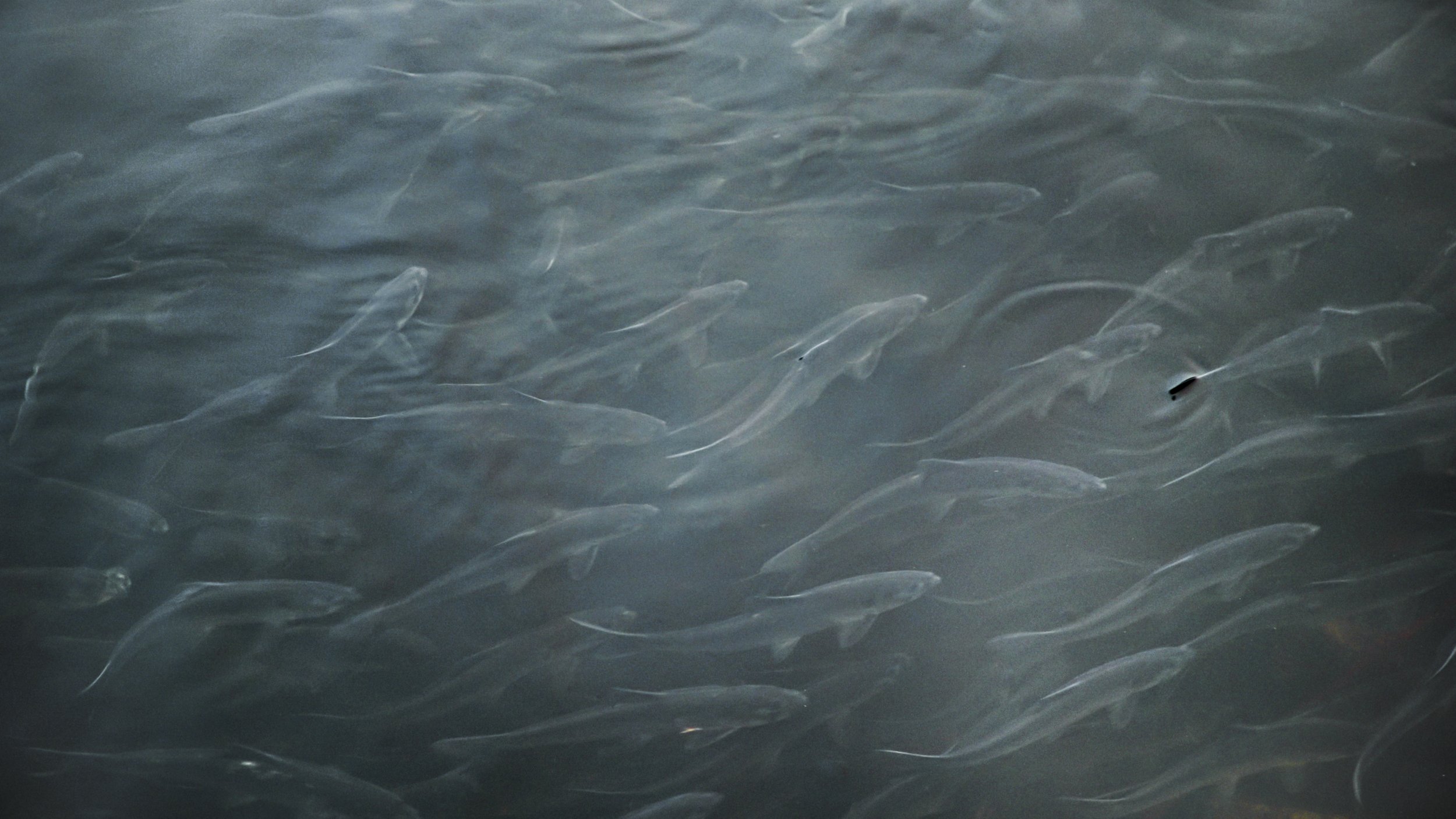A captivating long, rectangular, panoramic illustration predominantly in shades of gray showcases a serene yet lively underwater scene. The image offers a unique view above and below the water's surface, depicting numerous sea creatures—possibly fish or sharks—swiftly swimming from left to right. A few fish deviate, moving upwards or in different directions, adding a dynamic touch to the scene. One shark's dorsal fin noticeably breaches the water's surface, creating subtle ripples that blend seamlessly with the faint highlights, possibly representing sunlight filtering through the surface. This intricate yet understated artwork masterfully captures the tranquil motion and vitality of marine life.